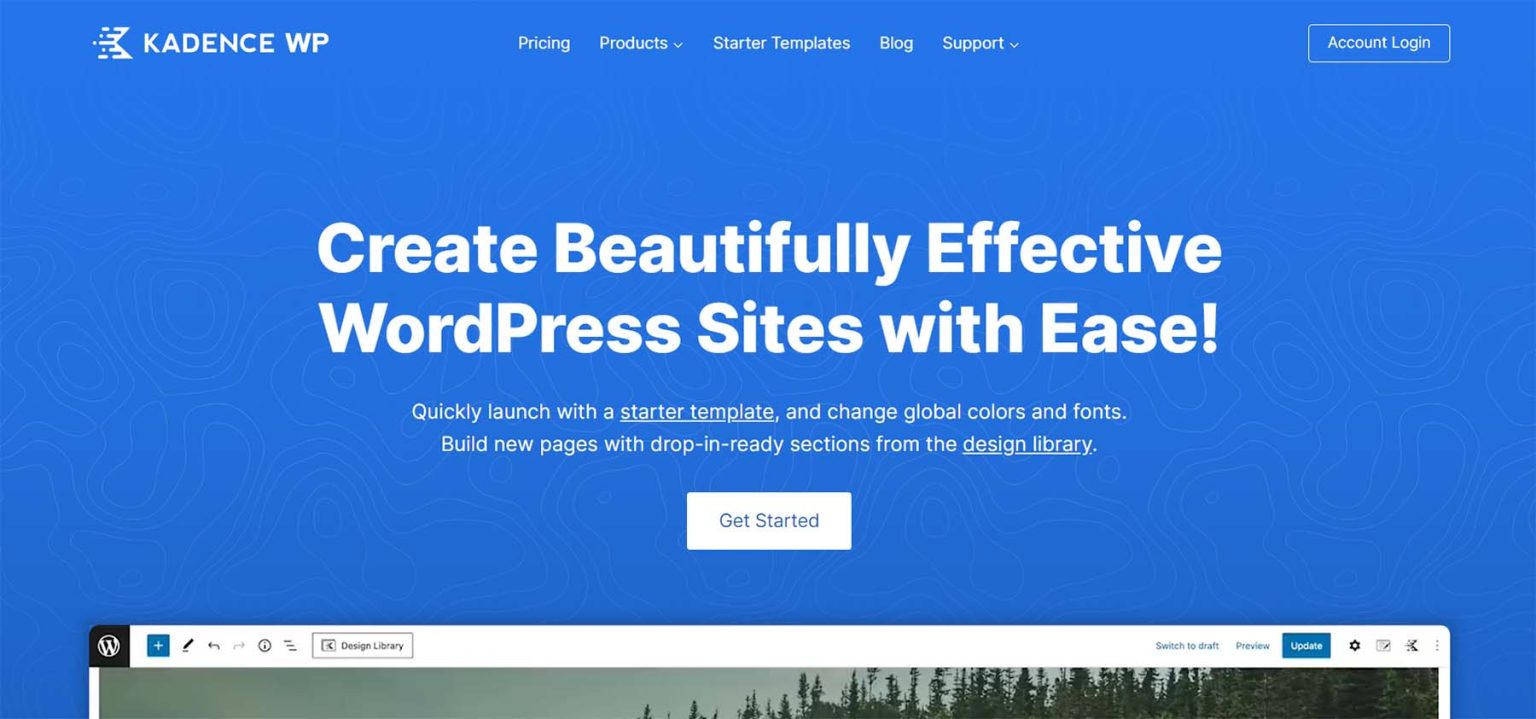Screenshot Description: This image is a screenshot showcasing the Candace W.P. website interface. The background is predominantly blue with white text, providing a visually appealing contrast. At the top of the screen, there is a navigation bar that includes options such as "Pricing," "Products," "Starter Templates," "Blog," and "Support." There are also links for "Account Login" and a prominent message: "Create Beautifully Effective WordPress Sites with Ease."

A central feature of the screenshot is a highlighted call-to-action to "Quickly launch with a Starter Template," where the phrase "Starter Template" is underlined, possibly indicating a hyperlink. Another notable feature is the instruction to "change global colors and fonts" and "build new pages with drop-in ready sections from the Design Library," with "Design Library" also underlined, hinting at another possible hyperlink.

In the lower portion of the screenshot, there is a "Get Started" button displayed in blue text with a white triangular icon next to it, encouraging users to begin their experience. Behind these elements, a computer screen is visible, depicting what appears to be a live representation of a website created using Candace W.P., reinforcing the ease and effectiveness of their WordPress site-building tools.